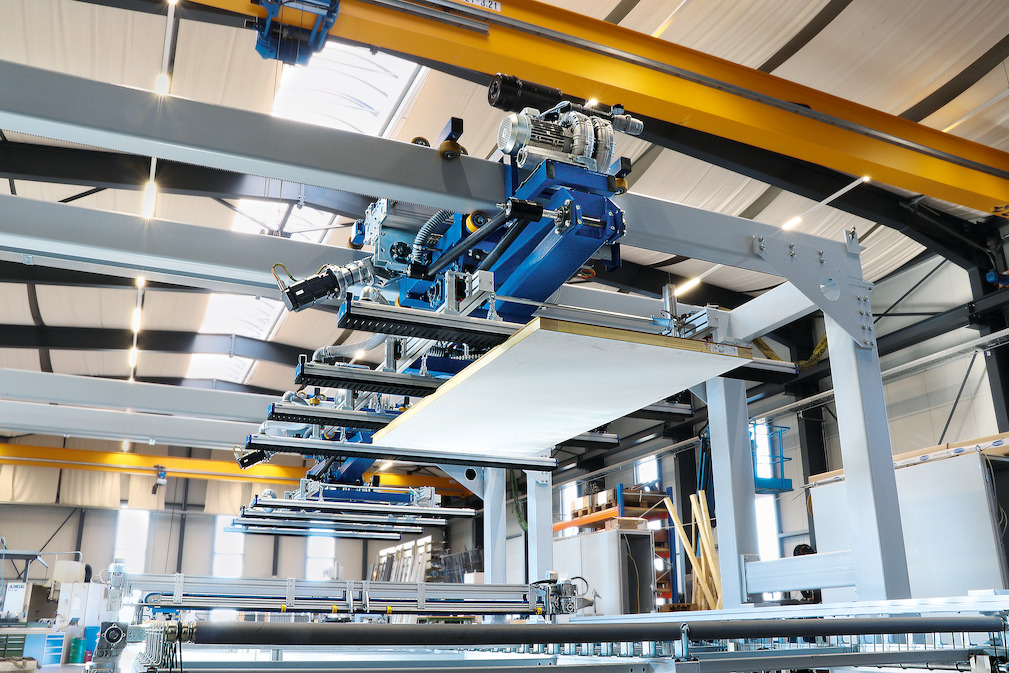This is a horizontally-aligned rectangular color photograph taken inside a large, modern, factory-like building, possibly corrugated steel, showcasing an elaborate assembly line setup. Dominating the scene are multiple vertical and horizontal gray metal frames supporting a blue apparatus, likely identifying or inspecting items on an assembly line below. The equipment has several long horizontal arms with fluorescent-style lights attached, each with a black bottom. Off to the sides and at the bottom of the image, more similar machinery can be seen. A notable feature is a suspended yellow metal bar extending diagonally from the upper right to the upper left of the picture. The ceiling appears to be white or beige sheet metal, well-lit, with some black beams and lights. The walls are unfinished, blending into the industrial aesthetic with hanging bars and vertical windows where light filters in. The colors present in the image primarily include light gray, blue, black, silver, and white. There are also silver motors, possibly electric, mounted on some equipment, and visible roller mechanisms at the bottom.